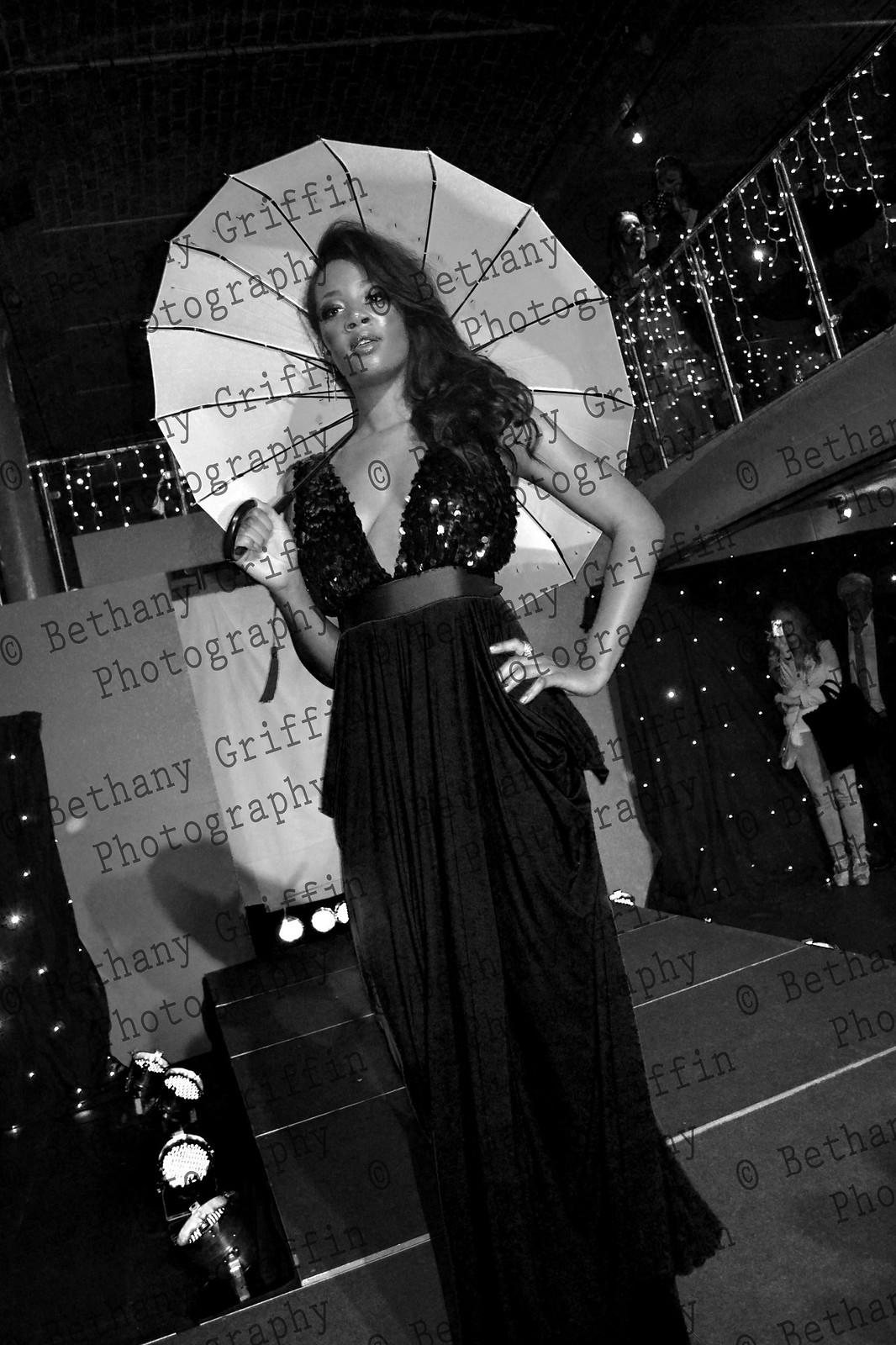In this striking black and white photograph, a woman stands confidently on a slightly tilted catwalk, posing dramatically. She's adorned in an elegant black gown featuring a deep V neckline embellished with sequins, which plunges to her waist, where a wide black belt cinches the dress. The skirt flows gracefully to the floor, likely made from a cotton jersey material, accentuating her poised figure. Her left hand holds an umbrella with its open canopy displayed behind her, while her right arm gracefully rests on her waist. The scene is set against a black background illuminated by twinkle lights and spotlights running down the sides of the runway, capturing the attention of an audience on the right. A watermark, "Bethany Griffin Photography," overlays the image, repeating diagonally from the bottom left to the top right, marking the artistry of the photographer.